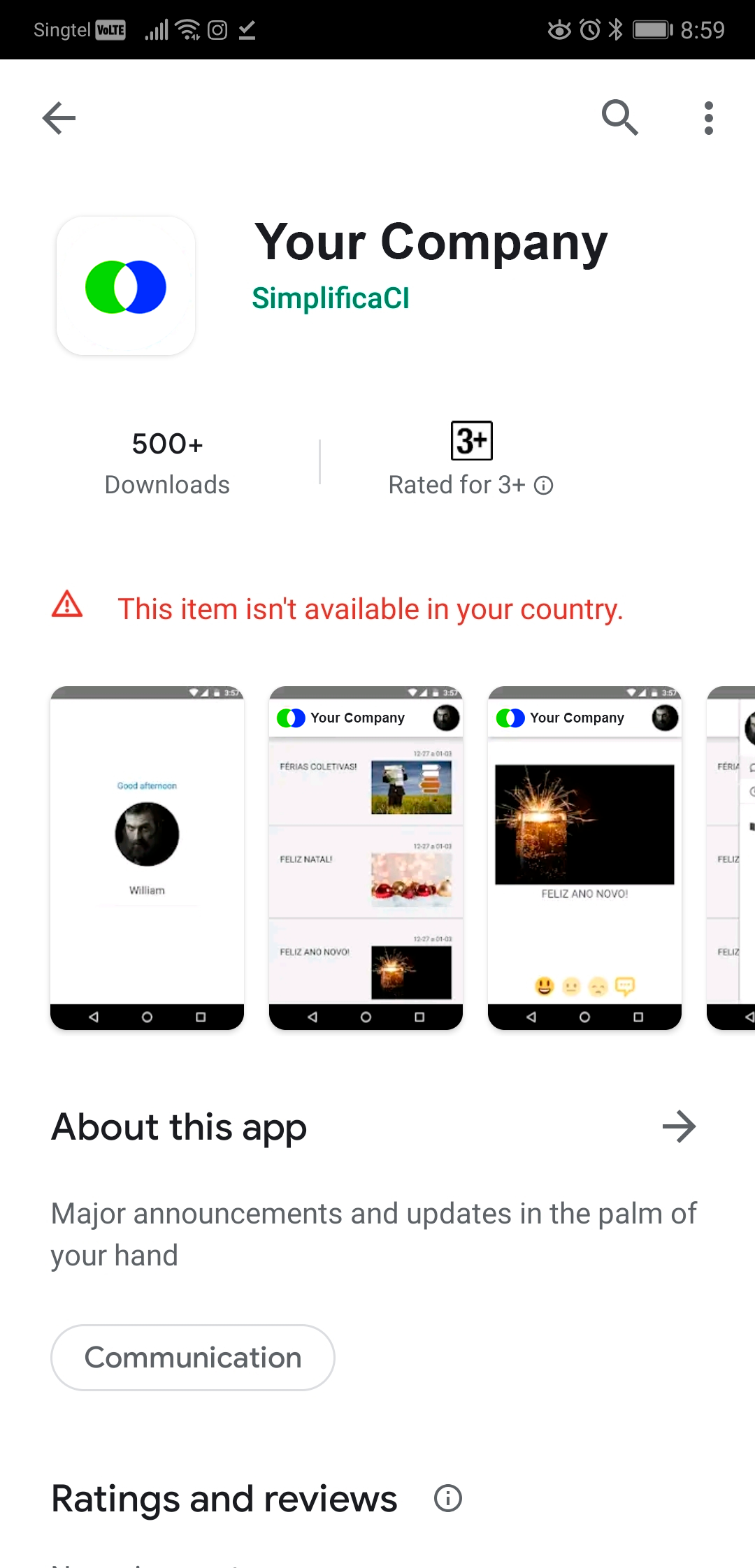Set against a white background, this image is a detailed screenshot of a mobile device. At the top, there is a black header displaying white text with the "Singtel" logo on the upper left, and a "VoLTE" indicator in a white box next to it. Icons indicate that Wi-Fi is connected with full reception bars. In the upper right corner, the time is shown as 8:59, with a fully charged battery icon beside it.

Dominating the screen below the header, "Your Company" is prominently displayed in large black text against the white background. Beneath this, "Simplifica CI" is noted in blue text. To the left of the text is an icon, which consists of a white square with two circles superimposed on it — one blue and one green, intersecting on the left side.

Further down, additional details include:
- A note indicating the app has "500+ downloads."
- A rating labeled for ages "3+."
- A red text warning stating, "This item isn't available in your country."

Following this, there are three images of tablets arranged from left to right. Below these images, a section header reads "About this app," prominently in bold black text.